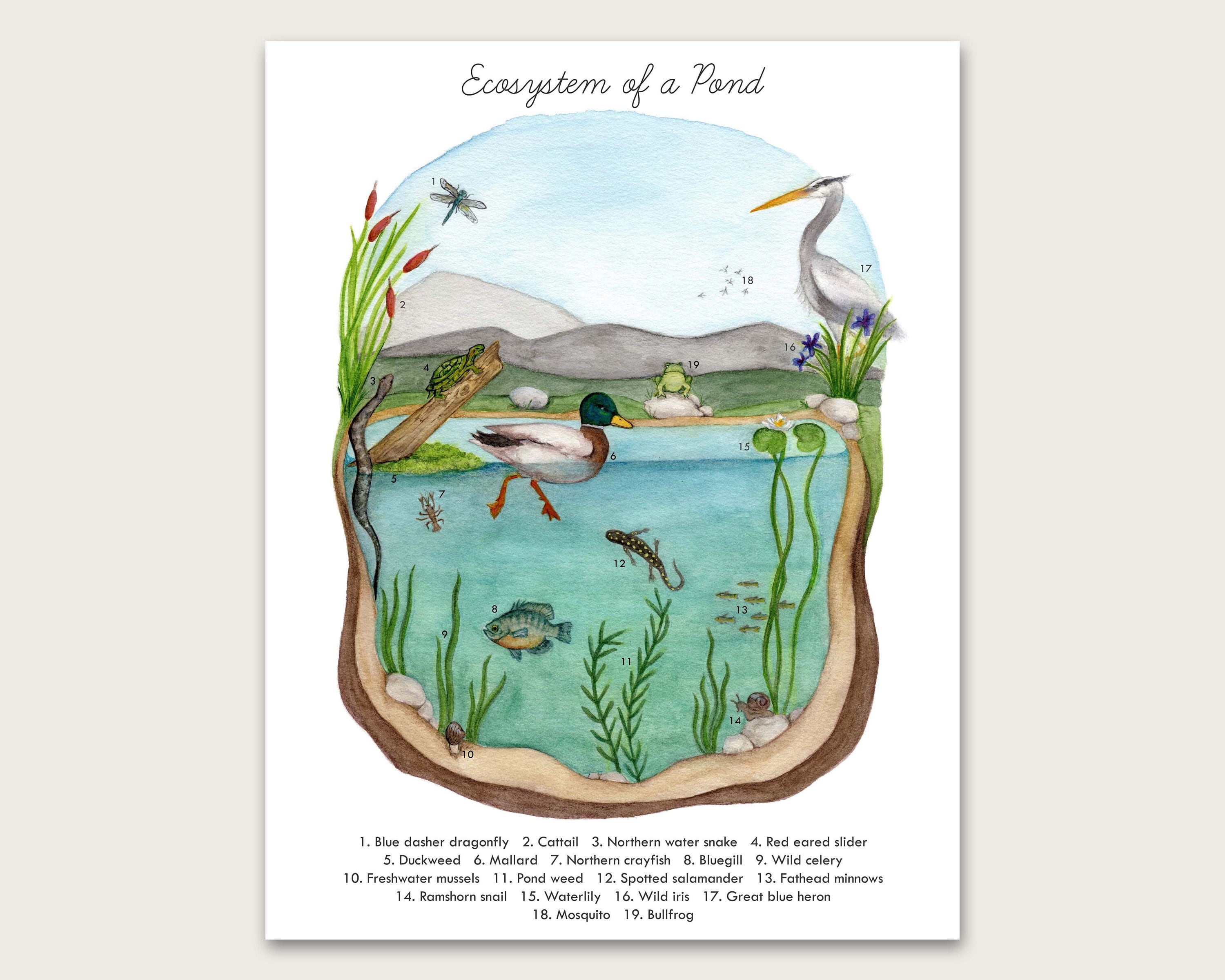The image depicts a detailed animated scene titled "Ecosystem of a Pond," set against a white cardstock background. At the top, the title is elegantly handwritten in cursive black. The centerpiece of the illustration is an oval depiction of a pond ecosystem bustling with life. The background features light blue, cloudy skies and distant mountains. On the left side, a tree branch extends over the scene, hosting a red-eared slider turtle and a northern water snake. Below, there's cattails and other plants at the pond's edge.

Within the pond's blue water, a vibrant array of aquatic life can be seen. A notable mallard duck with a green head, white body, and brown-tipped wings is prominent, half-submerged in the water. Various fish, including bluegill and fathead minnows with distinct blue and yellow coloring, swim beneath the surface. A brown-spotted salamander and a ramshorn snail are visible among the aquatic plants, such as wild celery, pondweed, and water lilies, which also include duckweed. 

Among the flora, irises and wildflowers add color around the shore. The center features a frog perched on a rock. A large shorebird, likely a great blue heron with a distinctive yellow beak, is seen standing nearby. Above the water, a dragonfly (Blue Dasher), a mosquito, and possibly a firefly or another insect hover in mid-air, contributing to the vibrant ecosystem. This detailed illustration serves as a comprehensive visual representation of the diverse and interconnected life found within a pond ecosystem.